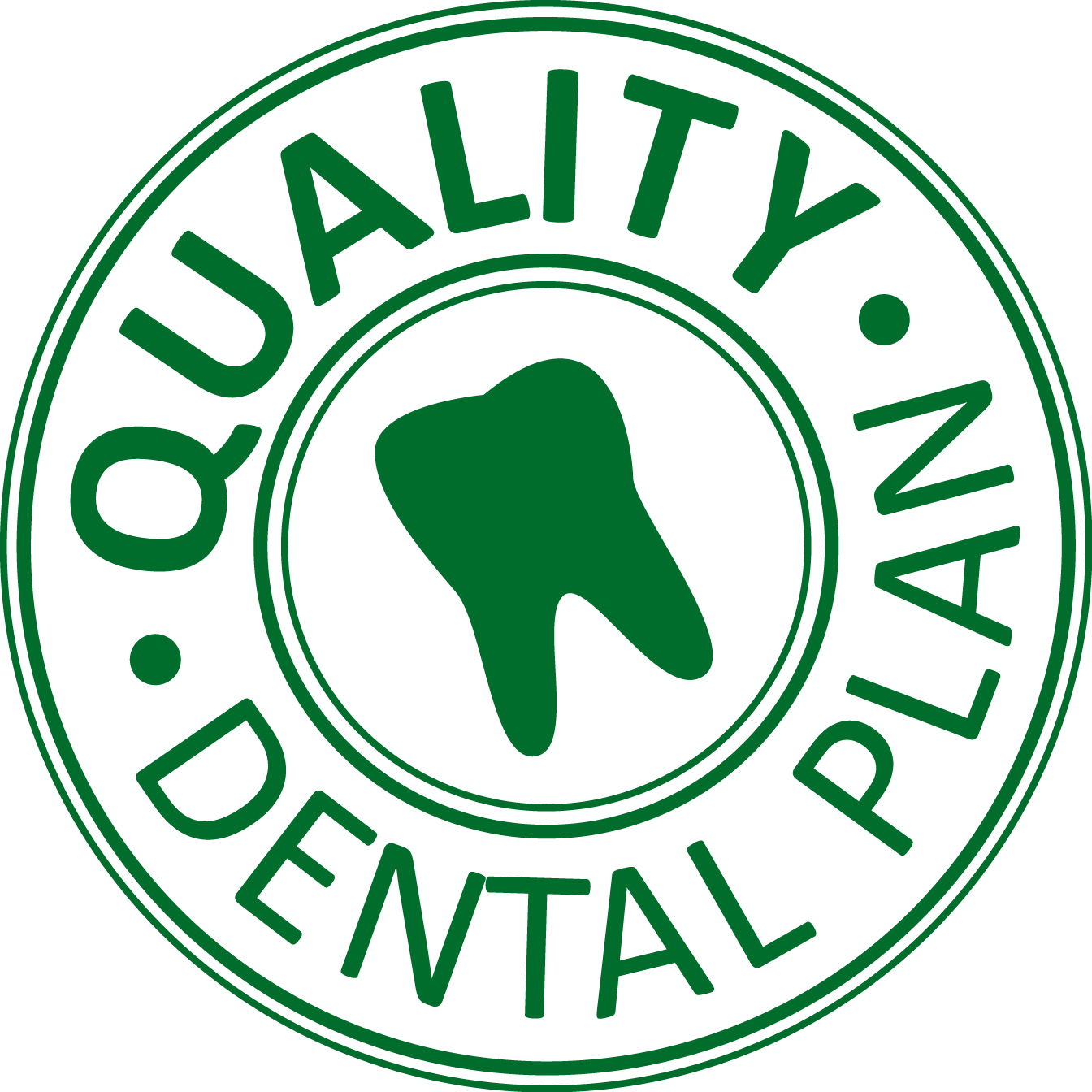The image showcases a minimalist circular logo for a dental company, predominantly using green and white colors. The background is completely white, providing contrast that highlights the green elements. The logo consists of several concentric circles: a large outer green circle featuring text, "Quality • Dental • Plan" in green font, slightly tilted to the left, with bullet points separating the words. Inside this outer circle is a slightly smaller bold green circle, followed by a white circular band, and then another bold green circle enclosing the central feature. At the heart of the logo is a smaller green circle containing a fully green, slightly tilted silhouette of a tooth. In total, there are four concentric circles, creating a layered, dimensional effect for the dental company logo.